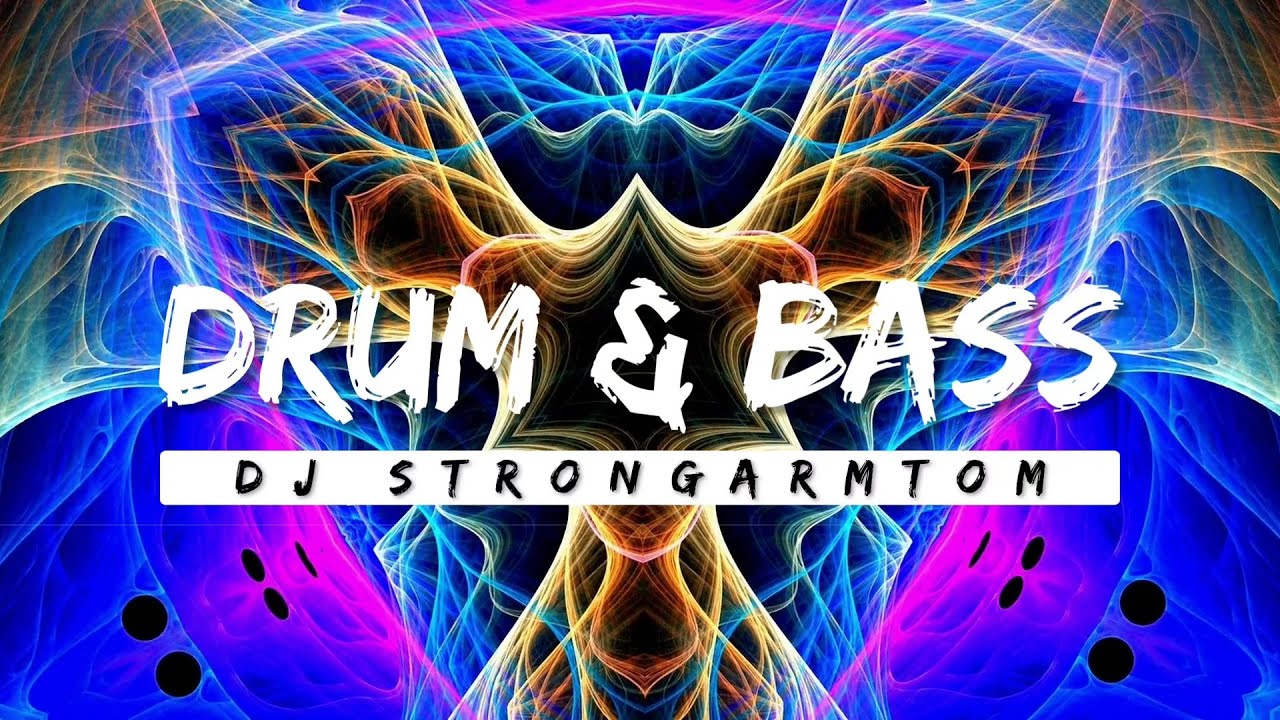This image depicts a vibrant advertisement for a Drum and Bass album or event, featuring DJ StrongArmton. The design is psychedelic and cartoonishly futuristic, perfectly capturing the dynamic energy of the music genre. The central figure, a girl with long hair, is illustrated with her hair transforming into a vivid, colorful aura reminiscent of static electricity globes, with strands of hair being pulled upward and outward. The background is a gradient of colors, starting with a black center that transitions to bright violet-purple edges. Various geometric and symmetrical lines and shapes in teal, blue, yellow, greens, and medium orange embellish the image, giving it a complex, layered appearance. The text "Drum and Bass" is prominently displayed in the foreground, with a white bar beneath it containing the stylized name "DJ StrongArmton." Overall, the visual elements merge to create an energetic and eye-catching promotion.